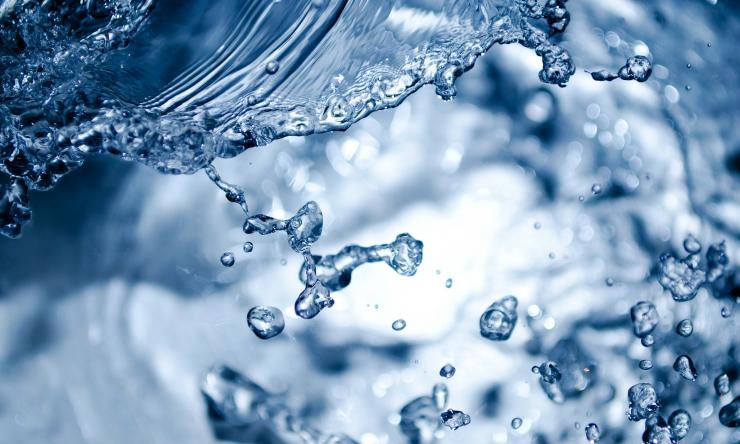A hyper-detailed close-up captures an intense splash of crystal-clear, blue-tinted water, possibly a professional photograph or a digital rendering. From the upper left, a wave-like cascade of water, as if poured from a glass, ripples across the image, with numerous droplets—varying in size from tiny spheres to larger oblong shapes—suspended mid-air. The foreground showcases these translucent droplets in impressive detail, some scattering downwards and some caught in motion, indicative of the dynamic energy of the splash. The background, awash in shades of slate blue, is deliberately out of focus, revealing blurred whorls and ripples that suggest more water, creating a reflective, overexposed center reminiscent of swirling currents beneath a choppy surface. Together, these elements combine to form a striking display of water's fluidity and motion, bursting with clarity and life.